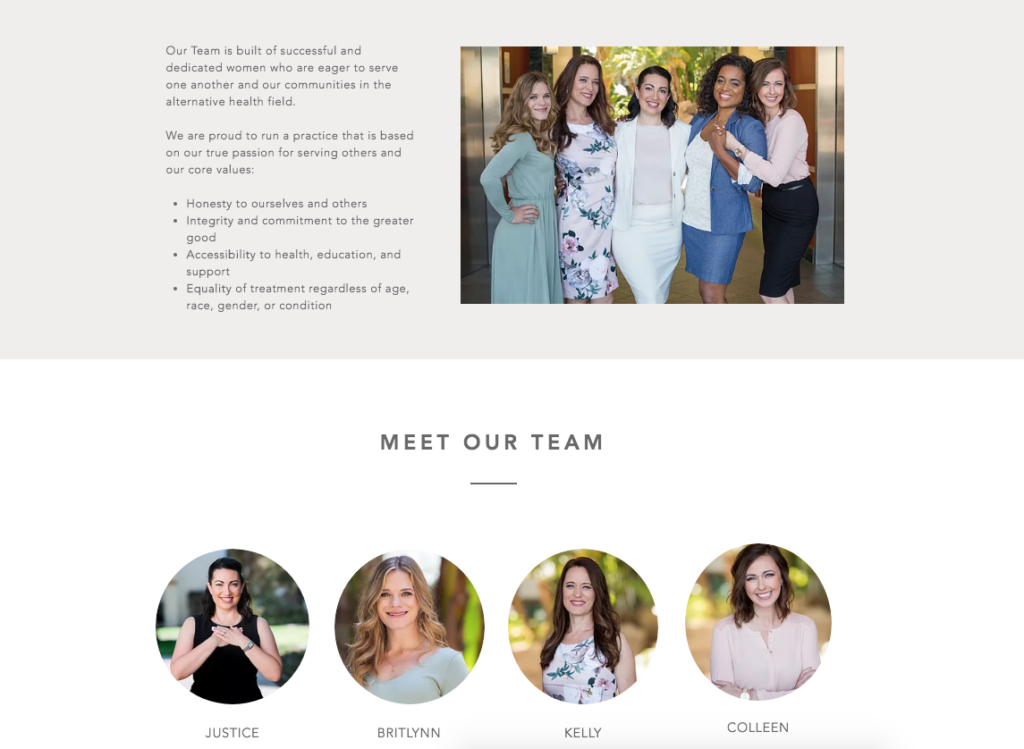The webpage introduces the company's dedicated team, focusing on their commitment to the alternative health field. 

At the top of the page, a prominent light gray rectangular border frames the content. Within this border, slightly skewed to the right but centrally aligned, is a photo featuring five professional women dressed in business attire, including dresses, skirts, and blazers. 

To the left of the photo, in black font, the text reads:  
“Our team is built of successful and dedicated women who are eager to serve one another and our communities in the alternative health field.”  
Beneath this, the text continues:  
“We are proud to run a practice that is based on our true passion for serving others and our core values.” 

Following this statement are four bullet points that outline the core values:
1. **Honesty to ourselves and others.**
2. **Integrity and commitment to the greater good.**
3. **Accessibility to health, education, and support.**
4. **Equality of treatment, regardless of age, race, gender, or condition.**

Below the gray rectangle, a white rectangular section houses the title "Meet Our Team" in black font, centered near the top. A small horizontal line, matching the length of the word "our," acts as a subtle separator below the title. 

Underneath this, four circular profile pictures of the team members are displayed, each accompanied by their name in black font. 

1. **Justice** - A brunette woman in her 30s, wearing a sleeveless black top. She is posed with her hands over her heart, exuding a sense of compassion and commitment. 
2. **Brittlyn** - A woman with shoulder-length curly dark blonde hair, in her late 20s, wearing a gray V-neck shirt. She is smiling warmly at the camera.
3. **Kelly** - A brunette woman in her late 20s or early 30s, with wavy brown hair that falls just past her shoulders. She is wearing a sleeveless white shirt with a floral print.
4. **Colleen** - A woman with dark brown, slightly wavy hair that reaches the top of her shoulders. She is wearing a white shirt with buttons, the top one casually unbuttoned, giving a relaxed and approachable appearance.

This detailed layout effectively introduces the team and their shared values, providing visitors with insight into their professional and personal dedication to the field of alternative health.